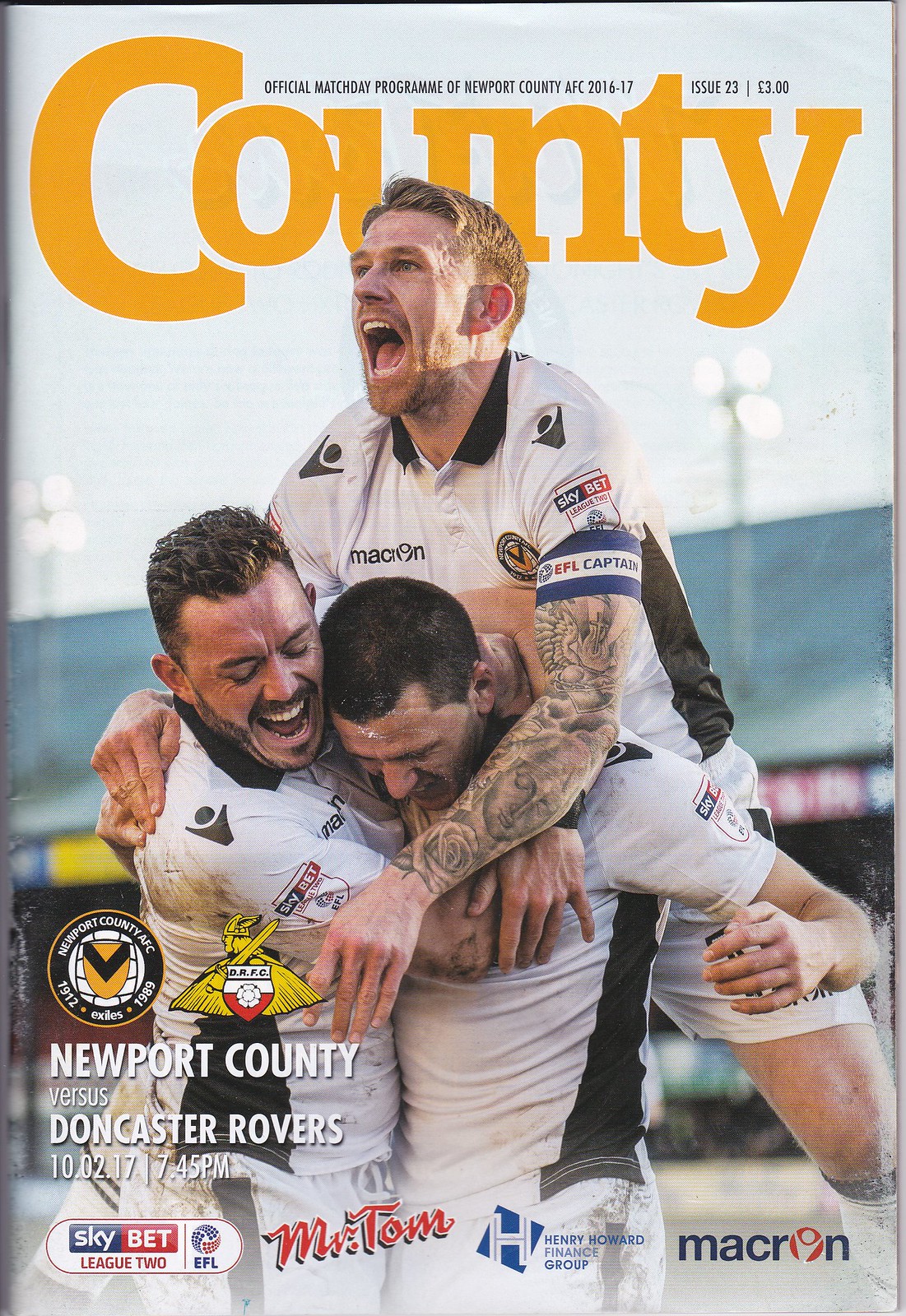The cover of the magazine "County" features a vibrant color photograph of three jubilant soccer players, evidently celebrating a significant moment, like scoring a goal or winning a match. This image captures the electric joy of the Newport County AFC team. The focal point is a player with short, orange-tinted hair, a stubbled beard, and a full arm sleeve tattoo on his left arm, who is caught mid-air, jubilantly jumping onto his teammates. He is screaming in excitement, embodying the triumphant spirit. All three players are donned in white jerseys with black accents, though one player's back is noticeably marked with dirt, suggesting an intense match. Above this spirited scene, the magazine title "County" is boldly emblazoned in large, orange text. Complementing the visual at the bottom left corner, the text reads: "Newport County vs. Doncaster Rovers, 10-02-17 at 7:45 p.m." surrounded by various logos and sponsorships such as Sky Bet, Macron, Mr. Tom, and Henry Howard Finance Group. This issue, marked as Issue 23 of the 2016-2017 official match day program, is priced at three pounds.